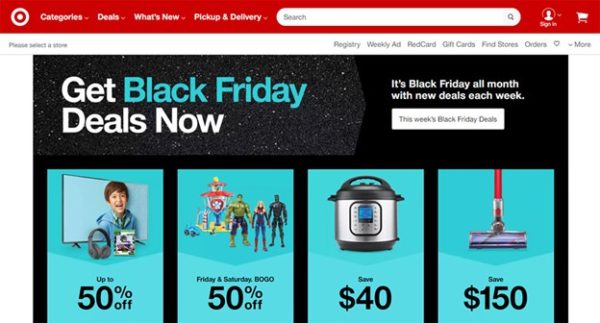The image displays a webpage layout predominantly themed in red and white. At the top, there is a red header containing the Target logo on the left side. Adjacent to the logo, there are several drop-down menus titled 'Category', 'Deals', 'What's New', and 'Pickup and Delivery'. To the right of these menus, a search box is prominently placed, followed by a 'Sign In' button, and a cart symbol to indicate shopping functionality.

Below this red header, a white box prompts users to select a store location. Following this prompt, there are additional options listed: 'Registry', 'Weekly Ad', 'Red Card', 'Gift Card', 'Find Stores', 'Orders', and 'More'.

Directly beneath this section, there is a banner text announcing, "Get Black Friday deals now!", with a smaller note on the right stating, "It's Black Friday all month with new deals each week."

The section below this announcement features another box labeled "This Week's Black Friday Deals". Within this box, there are four light blue sub-sections. The sub-section on the right illustrates a broom or mop, highlighting a deal that offers savings of $150.